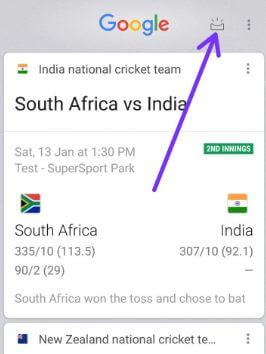Here is the cleaned-up and detailed caption:

---
Screenshot showing the Google search results page for the scores of the cricket match between South Africa and India. At the top center, the Google logo is prominently displayed. To its right, an icon resembling a crown can be seen, followed by a vertical ellipsis (three dots). An large blue arrow points upward from the middle of the screen towards the crown-like icon. 

The background is a gradient gray, transitioning into a white box that contains the match details. The title on the left reads, "Indian national cricket team." Below this, in a larger font, it states, "South Africa versus India." The date and time of the ongoing match are listed as "Saturday, 13th of January at 1:30 PM" at Tes SuperSport Park. The current status mentions that the game is in the second inning.

South Africa's score is recorded as "335/10 in 113.5 overs," and India's score is displayed as "307/10 in 92.1 overs." South Africa won the toss and chose to bat. The next line appears to show details for New Zealand's national cricket team, but the information is cut off and not fully visible in the screenshot.